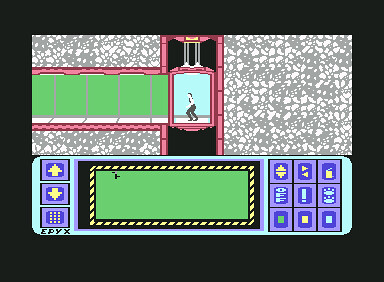This image resembles a nostalgic screen from an old-school handheld Game Boy game. On the left and right sides of the screen, there are up and down arrow icons, likely representing directional controls. The interface is organized into three distinct rows: the top row features yellow symbols, the middle row displays light blue symbols, and the bottom row consists of green, yellow, and blue symbols. While the exact function of these symbols is unclear, they evidently serve as control inputs for the game.

Centrally positioned between the directional arrows and the symbol rows is a rectangular frame, inside which is another smaller green rectangle bordered by a yellow-black striped pattern, possibly indicating a highlighted or active selection area.

Above this control panel, a character is depicted descending an elevator shaft into a green-colored hallway, suggesting a scene from the game’s adventure or exploration aspect. The overall aesthetic is undoubtedly retro, evoking the vintage appeal of classic handheld gaming, albeit with a simplistic and possibly monotonous design.